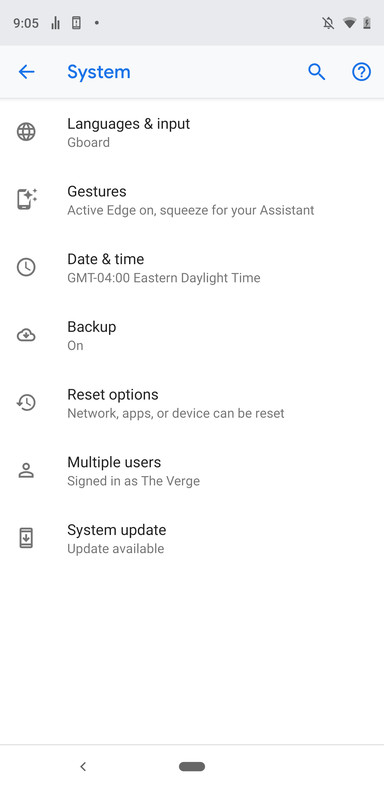The image showcases various screenshots of an Android device's system settings page. In the status bar at the top left, the time is displayed as 9:05. The network signal strength indicator is also visible. On the top right, you can see the Wi-Fi signal strength icon, the battery charging indicator, and the Do Not Disturb icon. The settings screen presents multiple system options, including "Languages and input," "Gestures," "Date & time," "Backup," and "Reset options." The page indicates that network, apps, or the device can be reset. It shows that multiple users, including a user named "Verge," are signed in. There is a notification for a system update being available. Additionally, the search icon and the help icon are located on the same screen. The "Backup" feature is turned on, and the date and time settings are configured to GMT-4 (Eastern Daylight Time).